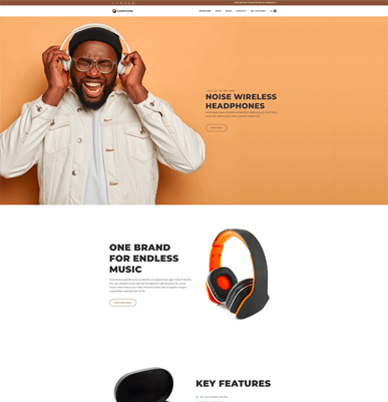The webpage prominently displays an advertisement for wireless headphones. At the top of the page, there is a vibrant orange graphic with bold text in the middle proclaiming "Noise Wireless Headphones." The secondary text, while present, is too small to read in this image. To the left of this text, a joyful Black man is depicted wearing the headphones. His mouth is wide open in a cheerful expression, eyes closed, as if he is immersed in his music. He is accessorized with glasses, a black beanie, a white bomber jacket, and a white shirt.

Below this main section, an enthusiastic tagline reads, "One Brand for Endless Music." Positioned next to the tagline is an image of the wireless headphones themselves. The headphones feature a sleek black exterior with a striking orange interior lining the ear cups. Further down, there is a partially visible black case, suggesting additional accessories or storage.

Towards the bottom of the page, the word "Features" stands out in large black letters against a clean white background, indicating where detailed product specifications might be listed.